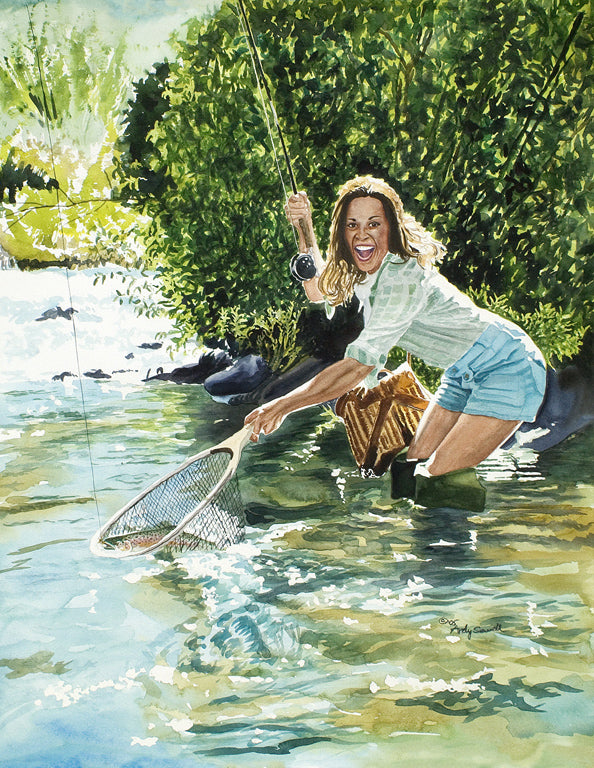In this watercolor illustration of muted colors, a woman stands joyfully in a small creek or river, looking directly at the viewer with a beaming smile. Her brownish hair falls just below her shoulders, and she wears a light blue blouse with rolled-up sleeves, tucked into faded blue cutoff shorts. She is up to her knees in water that shows hues of light blue and light brown. The woman holds a fishing net in her left hand, containing a fairly good-sized fish, while her right hand grips a fly fishing rod with a string leading out of the frame. She also wears wading boots that reach mid-thigh. Behind her, a bushy landscape featuring olive and pine green trees, along with some rocks, adds depth to the scene. A bag, possibly a lunch bag, can be seen behind her, and a large tree dominates the right half of the background. The water in the distance appears to flow downstream into rapids. Her expressive face with an open mouth conveys excitement and happiness at her successful catch.